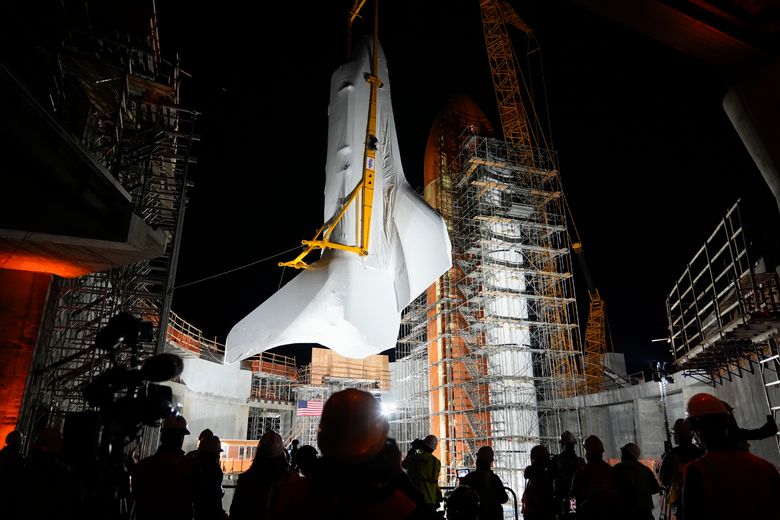In the midst of the dark night sky, an intricate scene of meticulous preparation for a space shuttle launch unfolds. At the center of the image stands the prominent space shuttle, its body enveloped in a protective white cloth. This shrouded shuttle is elevated, held securely by vibrant yellow straps suspended from a crane, indicating ongoing assembly rather than immediate launch readiness. Flanking the shuttle on the right is an extensive metal framework with staircases winding their way upwards, reminiscent of scaffolding at a busy construction site. 

An imposing large orange crane and various construction elements, including grayish walls being assembled around the base, emphasize the industrious activity. Illuminating the scene, bright lights focus on the shuttle, contrasting starkly with the pitch-black sky. Silhouetted against this backdrop, a diverse group of individuals, some equipped with construction hats, keenly observes the progress, many capturing photographs of the iconic symbol of space exploration. Adding a touch of patriotism, an American flag, adorned in red, white, and blue, is visible in the background. The image, a blend of human effort, construction, and aspiration, captures a pivotal moment in the journey towards space.